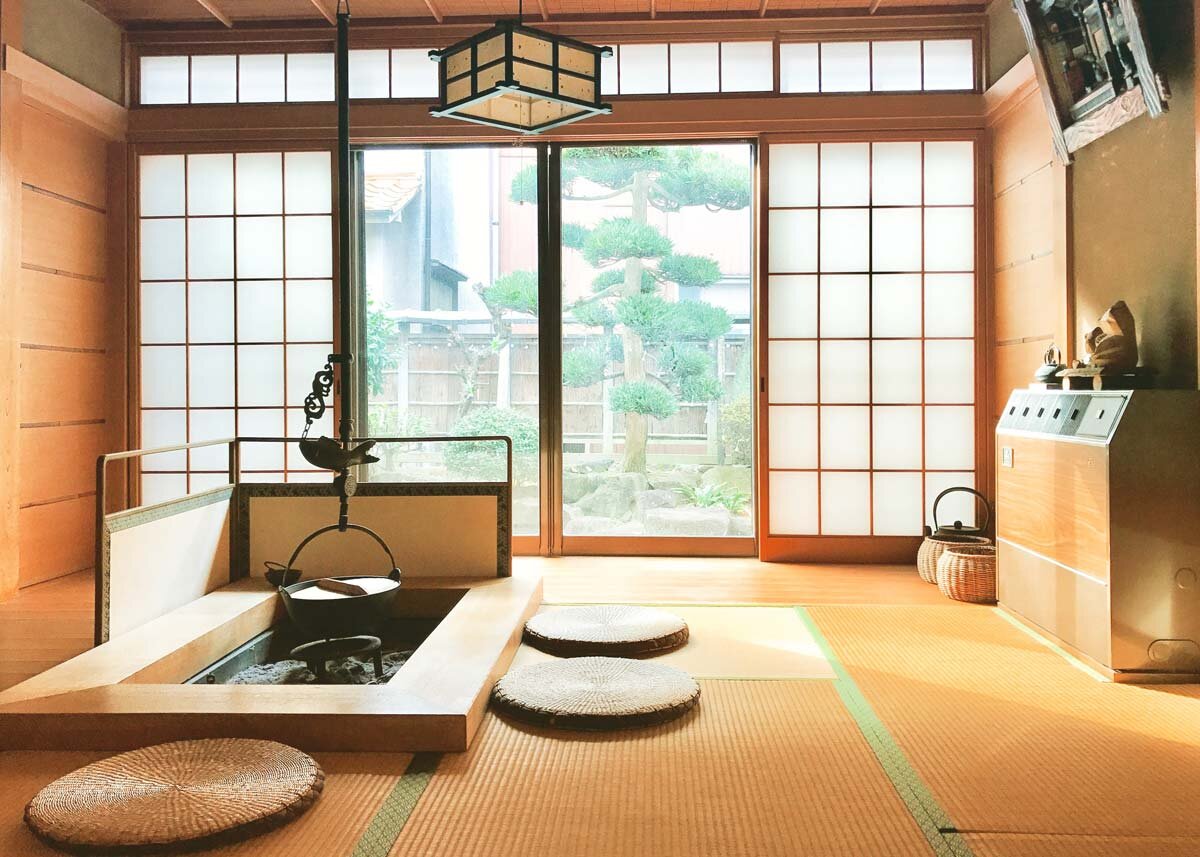In this detailed depiction of an Eastern-style, room, the space is characterized by its traditional Japanese aesthetic. Light brown wooden panels adorn the walls and ceiling, creating a warm and inviting ambiance. The room features a sliding glass door on the back wall, segmented into a grid pattern by white frames, allowing natural light to filter through their translucent paper panels.

Central to the room is an open rectangular fire pit, bordered by a light wooden frame that complements the overall decor. A cast-iron pot, with a slightly archaic design, hangs from a dark-colored pole descending from the ceiling, its position adjustable by an attached hook device. Surrounding the pit are three circular mats, woven from straw and featuring subtle green borders, serving as seating cushions.

On the right side, a cabinet rests against the wall, its lower section fitted with wicker baskets, adding to the room’s rustic charm. Above, a cube-shaped lantern dangles from the ceiling, framed in green with yellow rectangles and an open bottom, casting a downward glow over the space.

Outside the sliding door, the scenery includes a meticulously maintained garden visible through the semi-transparent doors. A Japanese maple tree stands prominent with its curvy, intricate trunk and lush green leaves, surrounded by a picket fence, another building, and a meticulously arranged assortment of gray rocks and green shrubs. This serene environment enhances the tranquil atmosphere inside the room.

Overall, the room blends modern elements with traditional Japanese décor, creating a space that feels both timeless and contemporary.